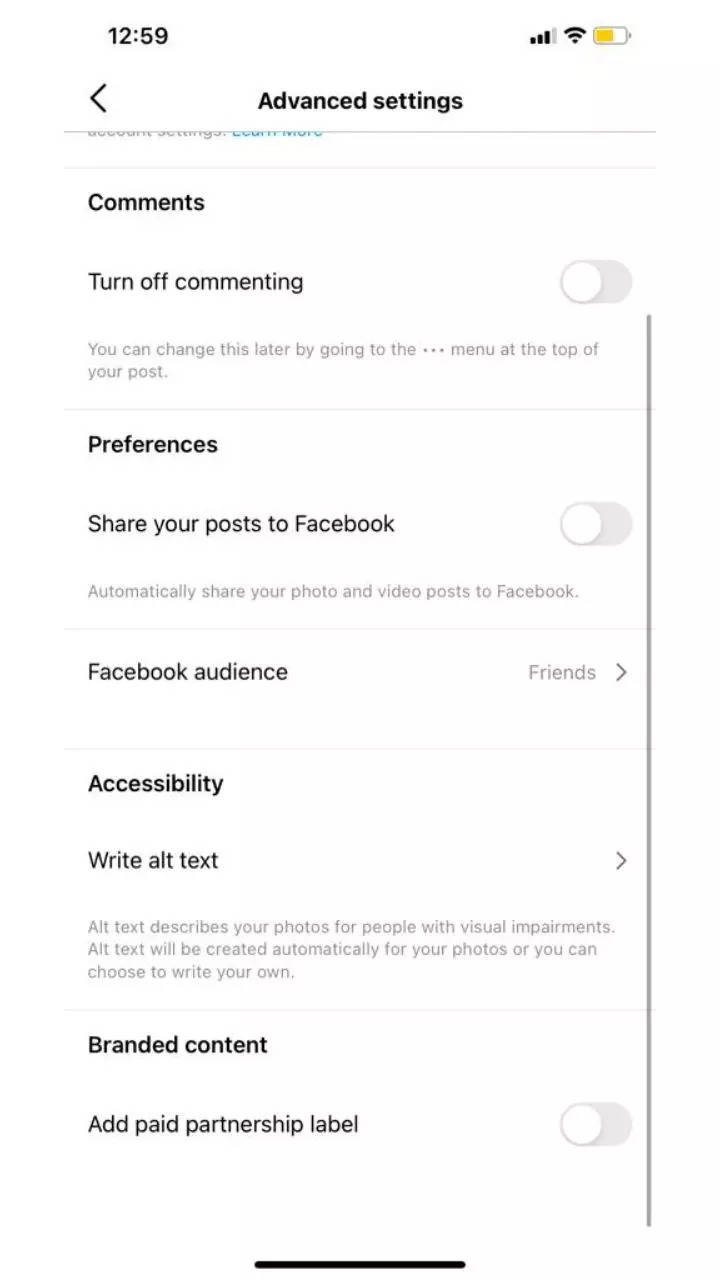This image is a screenshot of a phone displaying its "Settings" section. At the very top, the time is shown as 12:59, and to the right, there are four signal bars with three highlighted, a Wi-Fi icon, and a battery icon indicating a bit more than half charge.

Below this top bar, there's a left-pointing arrow on the left side. Centered at the top of the screen, it reads "Advanced Settings." Directly beneath this title, on the left, the word "Comments" is displayed, followed by an option labeled "Turn off commenting" with a toggle switch that is currently off.

A line of text below reads, "You can change this later by going to the ... menu at the top of your post." Following this, the "Preferences" section appears.

Within "Preferences," there is an option labeled "Share your post to Facebook" with a toggle switch set to off. Below it, the text "Automatically share your photo and video post to Facebook" is shown, followed by a line separator.

Under the line separator, it reads "Facebook Audience" with a right-pointing arrow and "Friends" next to it. Another section below labeled "Accessibility" includes an option "Write Alt Text" also accompanied by a right-pointing arrow.

At the bottom, a body paragraph precedes the "Brand Collaboration" section. This section includes an option "Add Paid Partnership Label" with a toggle switch set to off.